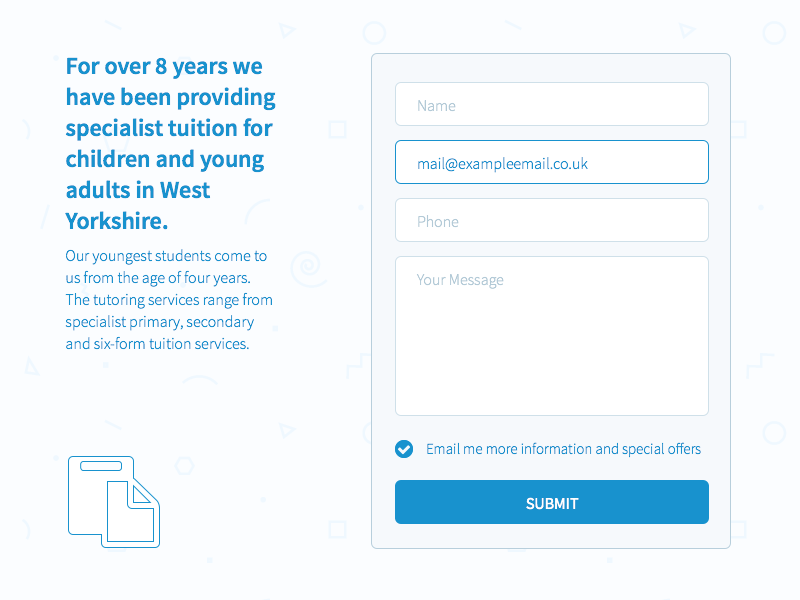Below is a refined and detailed caption for the described image: 

---

The image showcases an informative webpage from a tutoring service provider in West Yorkshire. On the far left side of the page, bold text asserts, "For over eight years we have been providing specialist tuition for children and young adults in West Yorkshire." Just below in a smaller font, it highlights that their youngest students start from the age of four years. The tutoring services span multiple educational stages including specialist, primary, secondary, and sixth form tuition.

On the right side of the page, there is a contact form designed for user inquiries. The form includes fields for entering your name, email, phone number, and a message. There is also an option to receive more information and special offers via email, which can be activated by ticking a checkbox. The 'Submit' button is conspicuously presented in blue, matching the predominant font color used throughout the image.